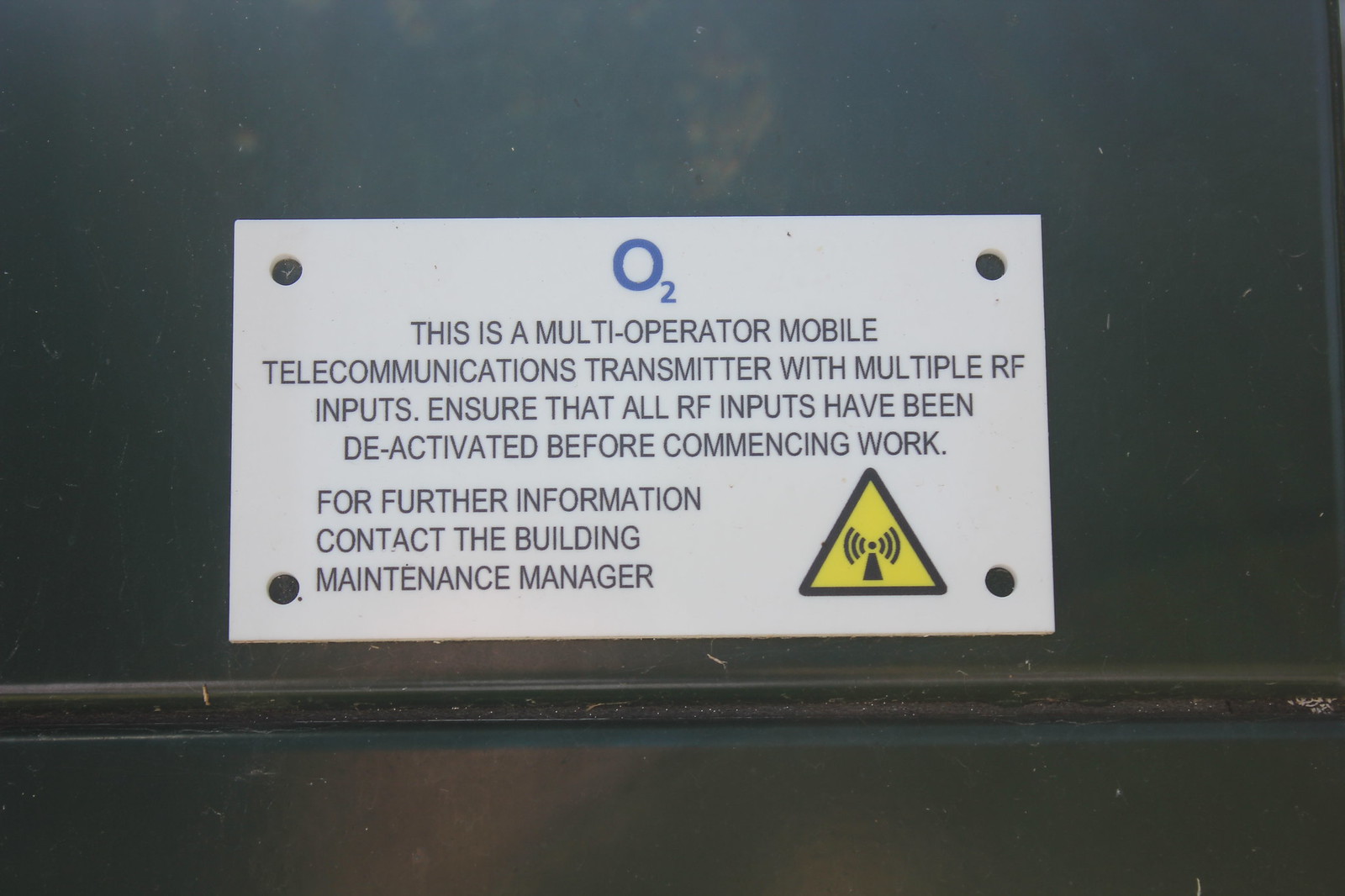The image depicts a metal plate affixed to a green piece of machinery. The plate is silver and secured with screws at each corner. At the top center, it has "O2" written in blue text. Below this, in black text, it reads: "This is a multi-operator mobile telecommunications transmitter with multiple RF inputs. Ensure that all RF inputs have been deactivated before commencing work. For further information, contact the building maintenance manager." In the bottom right corner, there is a yellow triangle with a black border, featuring an icon of a device transmitting radio waves.